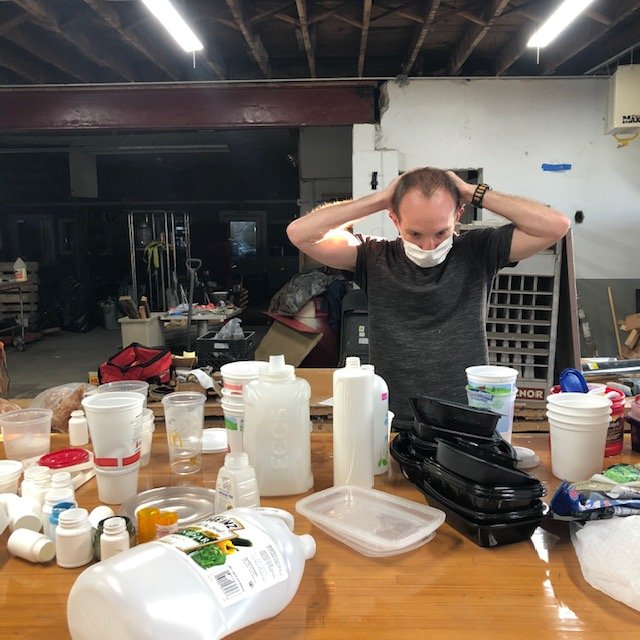In the image, a man with a light skin tone, wearing a black T-shirt and a white face mask, stands at a light brown wooden table cluttered with various objects. His hands are positioned behind his head, and he has a bracelet on his left wrist. His hair appears to be a lighter brown shade. The table is covered with numerous items, including jugs, white and black plastic tubs with clear lids, and a few glass and plastic containers. There is also a white five-gallon bucket on the table.

The background reveals a white wall on the right side and a metal roof, which looks aged and rusted in places. The roof is equipped with two rectangular white lights. Behind the man, there is a brown over archway and various pieces of equipment, including metal pipes. On the far left of the image, there appears to be a door with a square-shaped window on it. The overall setting seems to be industrial or a workshop of some kind, suggesting an atmosphere of diligent activity.